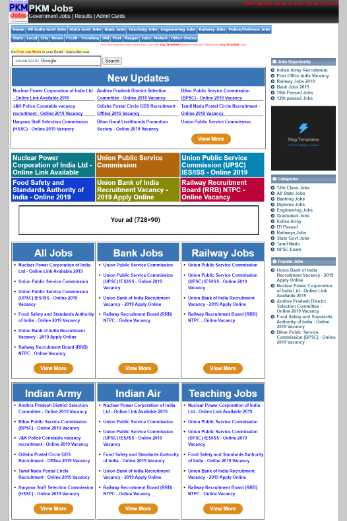The image is a vertically elongated screenshot of an outdated website, approximately twice as tall as it is wide. The text within the image is notably small, making it difficult to read due to the extensive content displayed. Both the left and right margins, roughly occupying 5-10% of the image each, are grey-colored.

In the upper left-hand corner, the text "PKM" is visible, styled in dark blue. Below this, there is a horizontal black bar extending across the width of the screenshot, featuring the white text "PKM Jobs." Directly beneath this bar, there is a line of text that is too small to decipher. 

The navigation area consists of a series of light to medium blue buttons with white text, though the specific text on these buttons is unreadable. Following this, there is a search box with an adjacent grey "Search" button on its right.

The website's overall aesthetic is reminiscent of late 1990s web design, characterized by basic colors, simple fonts, and minimal graphics. The design is blocky and lacks the sophisticated visual elements common in contemporary websites. There is nothing flashy or modern about it, revealing its vintage origins.